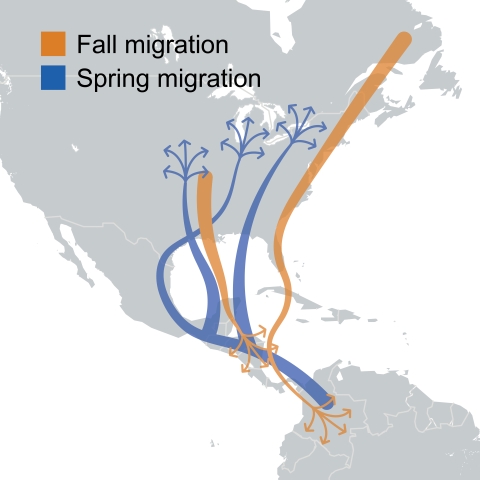This image is a detailed graphic representation of bird migration patterns across North and South America, depicted in shades of grey against a white background. The map includes a legend with orange indicating the Fall Migration and blue for the Spring Migration. The routes are illustrated as bands with small arrows indicating direction.

For the Spring Migration, the blue band originates from the top right corner of South America, traverses Central America, and extends into Mexico, branching into three main routes across North America, each with five distinct arrows showing subdivided paths.

The Fall Migration, shown in orange, starts from the top right of the image above Nova Scotia in Canada. One route travels down the East Coast, passing Florida and Cuba, wraps around Central America, and extends into South America with three to four offshoots. Another route begins in the Midwest United States, crosses the Gulf of Mexico near New Orleans, and concludes with branches in Central America.

This highly detailed graphic provides an overhead view and serves as an informative tool for understanding the seasonal migration patterns of birds across the Americas. The legend in the image clearly indicates the Fall and Spring migrations, enhancing the comprehension of these intricate pathways.